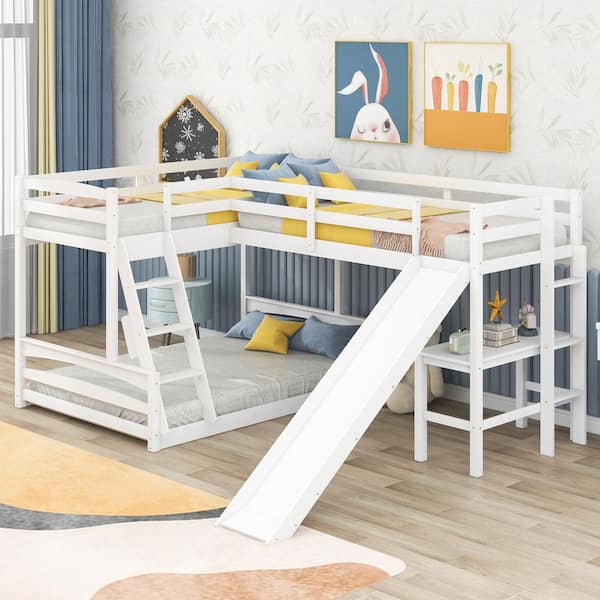The image depicts a meticulously arranged children's room with a set of distinctive white bunk beds as the focal point. Situated on a hardwood floor of a light almond hue, the room features a multicolored rug in the lower left corner, displaying shades of yellow, black, white, orange, and green. This rug extends slightly into the room and contrasts beautifully with the wood flooring. 

The bunk beds are intricately designed: a lower bed that nearly rests on the floor, presumably a double bed, is positioned with its foot on the left and head against the wall. Perpendicular to this lower bed, an upper twin bed is accessible by a small white ladder placed on the bottom right. Adjacent to the lower bed, another twin bed lofts overhead, extending along the right side of the room and featuring a white slide that descends towards the colorful rug.

On the wall behind the beds, light-colored wallpaper with subtle designs enhances the room's aesthetic. Affixed to this wall are three whimsical decorations: a cartoonish portrait of a winking bunny, and an illustration of five differently colored carrots partially buried in the ground—depicting blue, yellow, and salmon hues. To the left-side wall, blue and white curtains frame a window, infusing the room with light. Additionally, a small white table with a few items sits under the bed on the right, completing the cozy and inviting atmosphere of this children's haven.